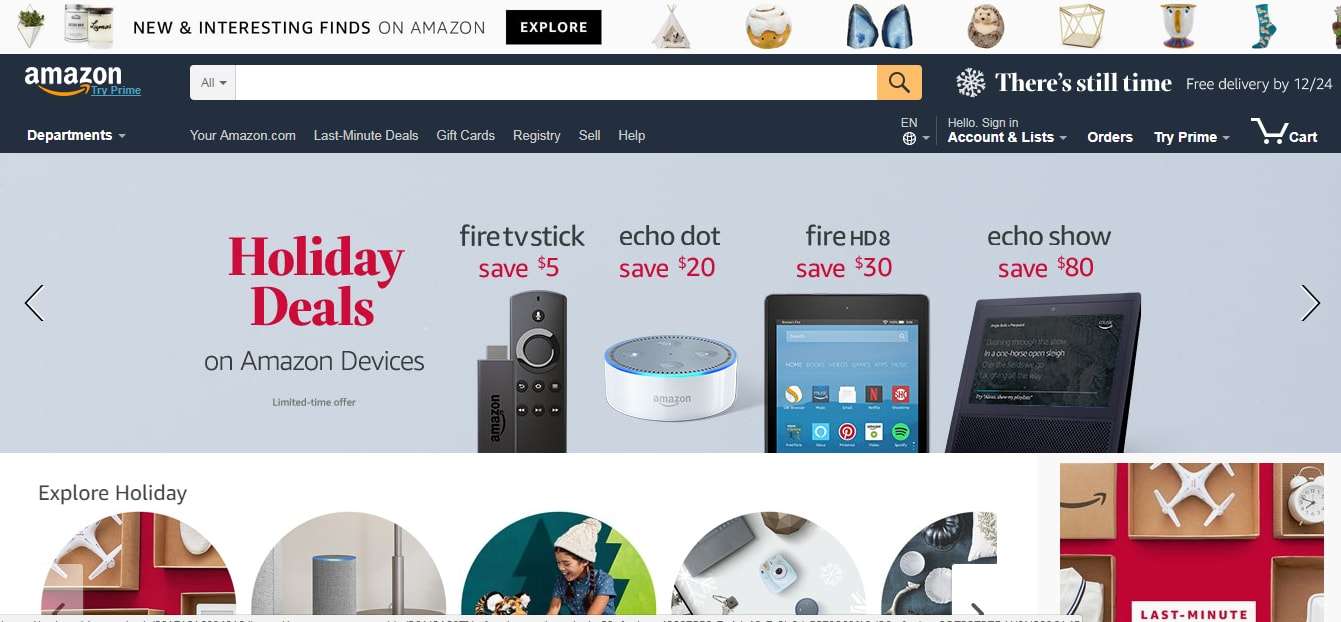The image is a multifaceted holiday promotion from Amazon, showcasing a variety of deals and products. 

In the top left corner, there's a section highlighting a new initiative by Amazon, set against a black background with an intriguing tint. Items featured include a cinnamon roll, a stone hedgehog figurine, and a teacup alongside a sock. The background has a festive theme with snowflakes and a reminder of last-minute delivery options by December 4th.

At the top center, there's an emphasis on Amazon's holiday deals, gift cards, registries, and customer service options. The navigation bar includes sections like "Sell," "Help," "Sign In," "Account & Lists," "Orders," "Prime," and "Cart." Specific deals are featured prominently: save $5 on Amazon devices, $20 on Fire TV Sticks, $30 on Fire HD 8, and $80 on other selected items.

Moving towards the bottom left, there's a holiday exploration theme, highlighting deals on a Bluetooth speaker and other tech gadgets. A person in a blue shirt and hat, with a light green background, is smiling, possibly indicating customer satisfaction. 

In the bottom center, you can see various items including a drone packaged inside a box, a traditional alarm clock with bells, an Amazon box displaying their iconic smile, and a necklace. The bottom right features a white and red motif with a brown box, adding to the festive display.

The composition effectively showcases a mix of holiday joy, tech gadgets, traditional gifts, and efficient delivery options, all aimed at enhancing the Amazon shopping experience during the festive season.